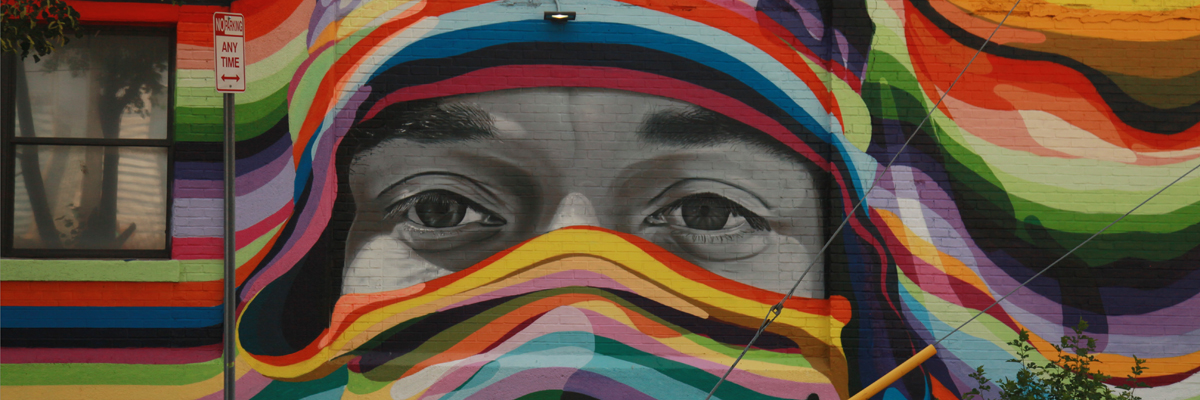This image showcases a vibrant and intricate mural on the side of a building, featuring a striking figure partially obscured by colorful, rainbow-hued cloth. The figure’s face is rendered in grayscale, encapsulating a profound gaze with prominently visible eyes and eyebrows, while the rest of the face is covered by the cloth. This headscarf-like covering resembles a hijab or a ski mask, draping down to conceal the bridge of the nose. The flowing lines of the scarf transition through various colors including red, yellow, orange, blue, light blue, green, and purple, creating a lively contrast against the monochromatic facial features. To the left of the mural, there is a black-trimmed window with an artistic depiction—seemingly of a tree in grayscale—painted on it, beyond which blinds are faintly visible. In front of the artwork, a "No Parking Anytime" sign stands prominently, accompanied by two wires with a yellow guard, adding to the urban streetscape captured in the image.